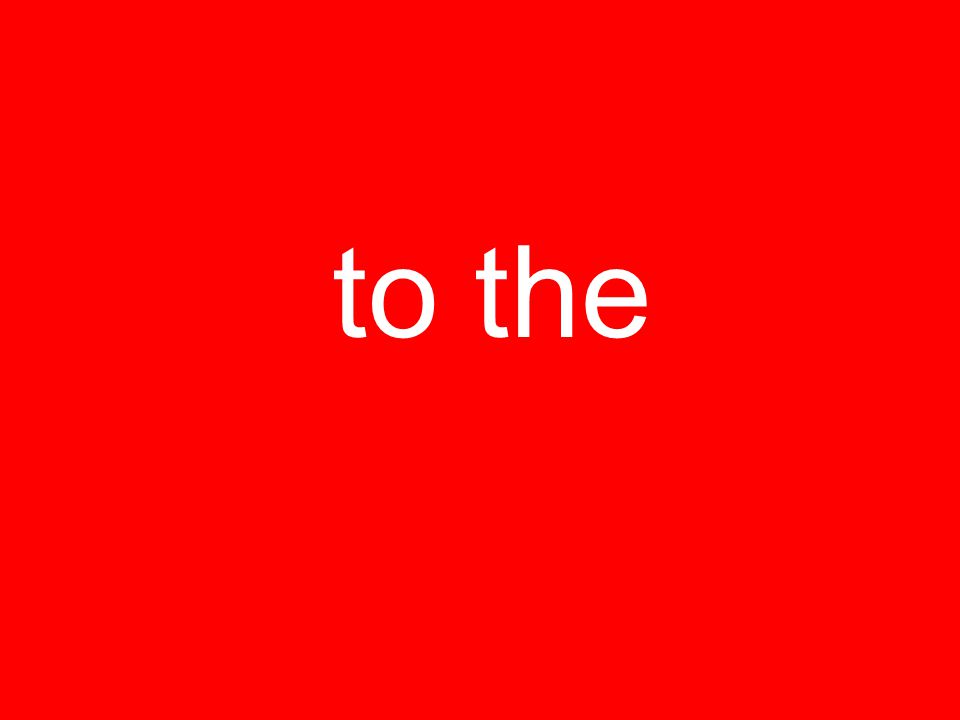The image features a solid red background with centrally aligned white text that reads "to the" in lowercase, sans-serif font. The text is positioned slightly above the vertical center of the image, taking up a single line of what would amount to six lines if the page were entirely filled. There are no additional objects or variations in color within the image; it is a stark and simple design that could be likened to a label or presentation slide. The red background encompasses the entire square image, providing a clean, uncluttered visual where the text stands out clearly.